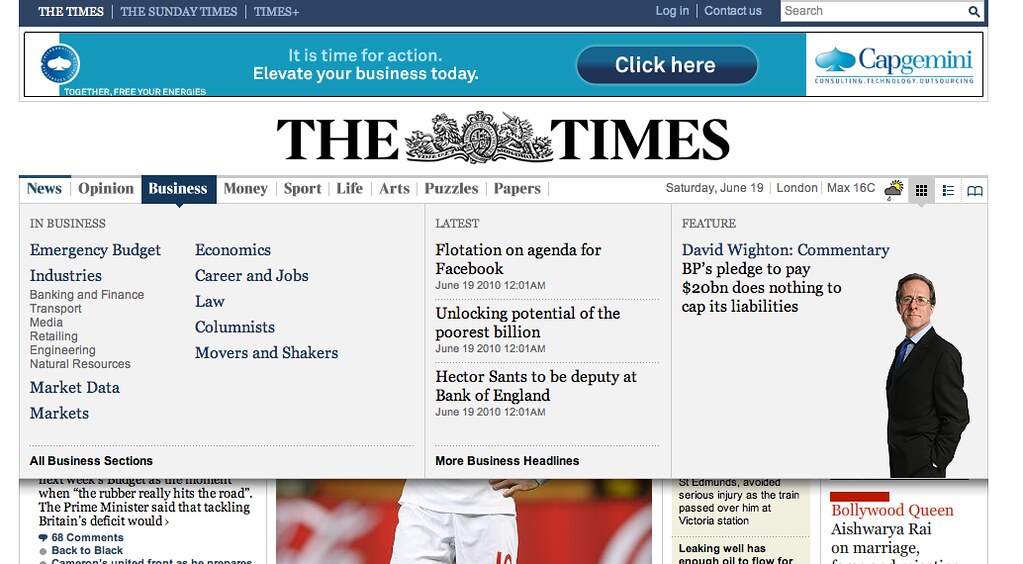The screenshot displays a webpage from a digital publication. At the top of the page is a dark blue banner. On the left side of the banner, in white uppercase letters, it reads "THE TIMES." A vertical white line separates this from "THE SUNDAY TIMES" in gray, which is followed by another gray vertical line and "TIMES+" in gray, with a plus sign on its right. On the far right side of the banner, in gray text, are the options "LOGIN," a vertical line, "CONTACT US," and a white search bar with a magnifying glass icon at the right end.

Below the banner is a rectangular section with a white left edge and an aqua-blue center. Straddling the line between white and blue on the left side is a dark blue circle featuring a white object inside. Centered within the aqua-blue section, in blue text, are the words "It is time for action." Beneath that, in white text, it reads "Elevate your business today." To the right side of this section is a blue oval button with the text "CLICK HERE," and further to the right is a logo reading "CAPGEMINI" in blue uppercase letters.

Centered below this section is the publication's name, "THE TIMES," in very large, bold, black letters, featuring an elaborate crest in the middle. Underneath this are the article headlines, preceded by a menu bar that lists various sections of the website: "News," "Opinion," "Business," "Money," "Sport," "Life," "Arts," "Puzzles," and "Papers." The "Business" section is highlighted in blue.

To the right of the headlines is a photograph of a man wearing glasses and a suit.